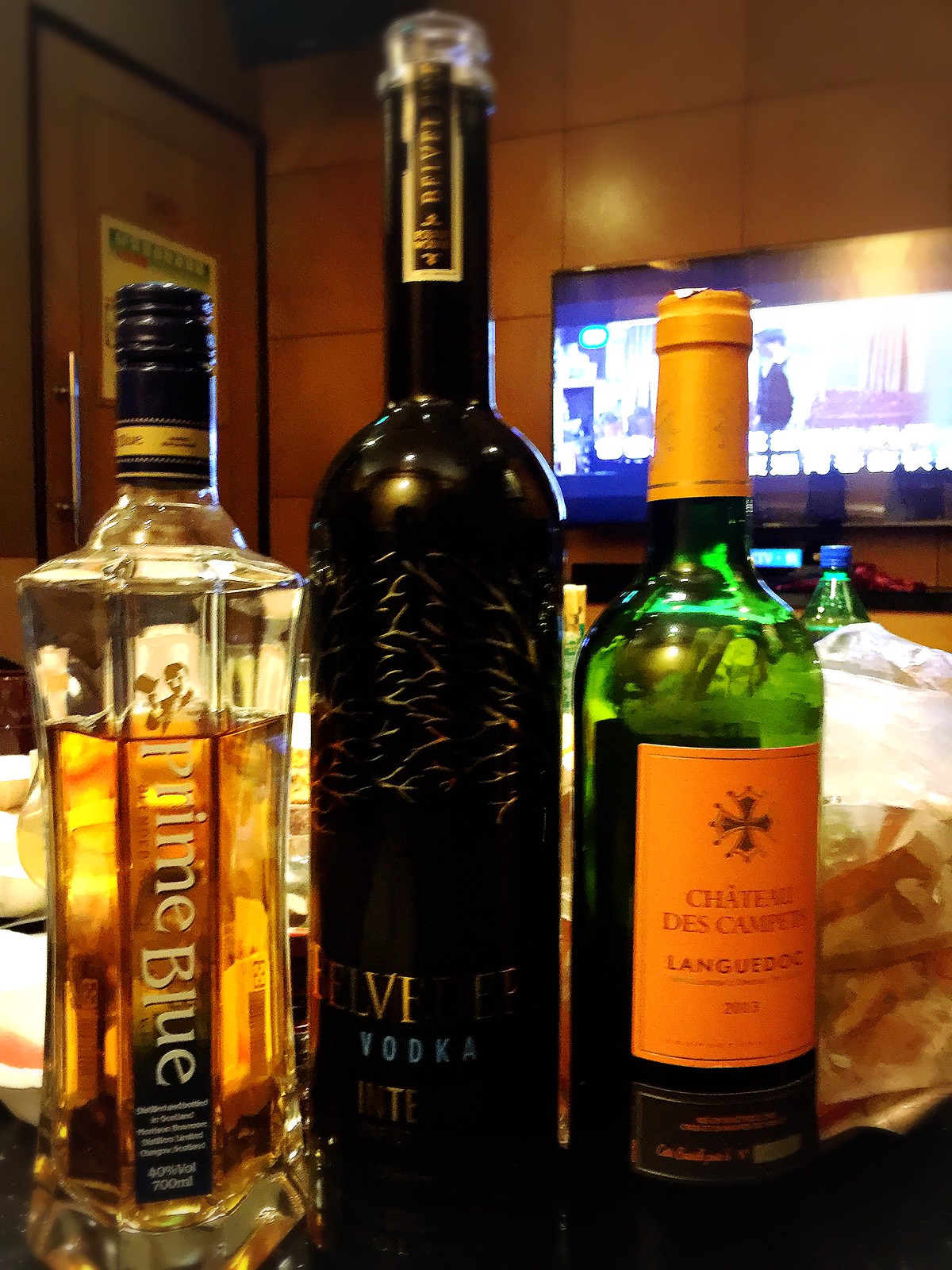The image features three distinctive bottles of alcohol prominently displayed on a wooden table. The first bottle on the left is Prime Blue, a whiskey with a clear glass bottle, a black cap, and about one-third of its contents already consumed. The bottle has an attractive design with the brand name written sideways. In the center stands the tallest bottle, a sleek black bottle labeled Elevate, identified as Belvedere vodka. Although the logo or brand is partially obscured by the angle, it features a design with tree branches. On the right is a green bottle of wine with French text that reads "Chateau des..." and has a yellowish-gold top. All three bottles have been opened and partially used, indicating they have been enjoyed. The background includes a door with a silver metal handle, a large screen TV turned on, and some white plastic bags and clutter scattered around, adding to the casual and personal atmosphere of the scene.